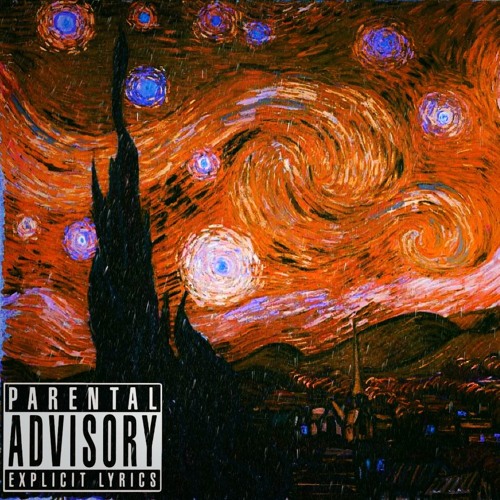The image is an album cover featuring a Parental Advisory Explicit Lyrics label in the bottom left corner, characterized by white text on a black background for "Parental" and "Explicit Lyrics," and black text on a silver background for "Advisory." The main artwork resembles Van Gogh's "A Starry Night," but with a bold color palette dominated by reds, yellows, and oranges, giving it an apocalyptic, expressionist vibe. Blue stars punctuate the swirled, fiery sky, and a dark, silhouette of a burnt-out tree or a building ascends into the heavens, adding to the dreamlike, almost oneiric quality of the scene. The bottom right features a village rendered in black and blue hues, under a sky that could be interpreted as either swirling in chaos or depicting a fiery volcanic event. This evocative cover blends elements of surrealism and expressionism, creating a haunting, visually striking image.